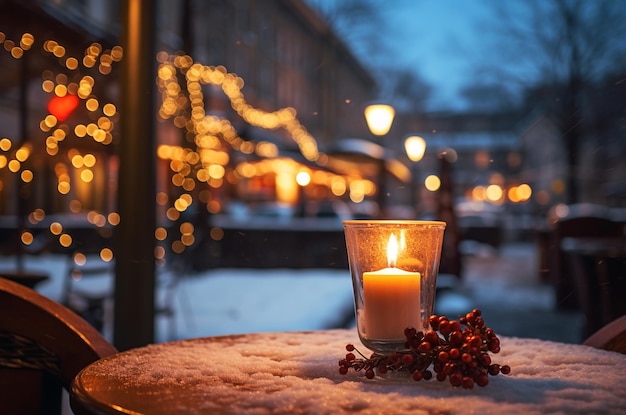A serene winter evening unfolds on an inviting outdoor patio. Centered on the table is an elegant glass-enclosed candle, softly illuminating its surroundings and casting a warm glow on an arrangement of berries scattered around its base. Snow delicately blankets the table and the ground in the distance, hinting at a recent snowfall. The backdrop features a charming commercial area with multi-story buildings, possibly containing apartments or a mall. In the distance, Christmas lights adorn storefronts, adding a festive touch to the scene. The overcast sky suggests the late evening hour, further emphasized by the gentle shine of the candlelight. The focus remains on the table and its intimate setting, while the softly blurred background includes two empty chairs, waiting patiently for occupants to enjoy this peaceful winter retreat.